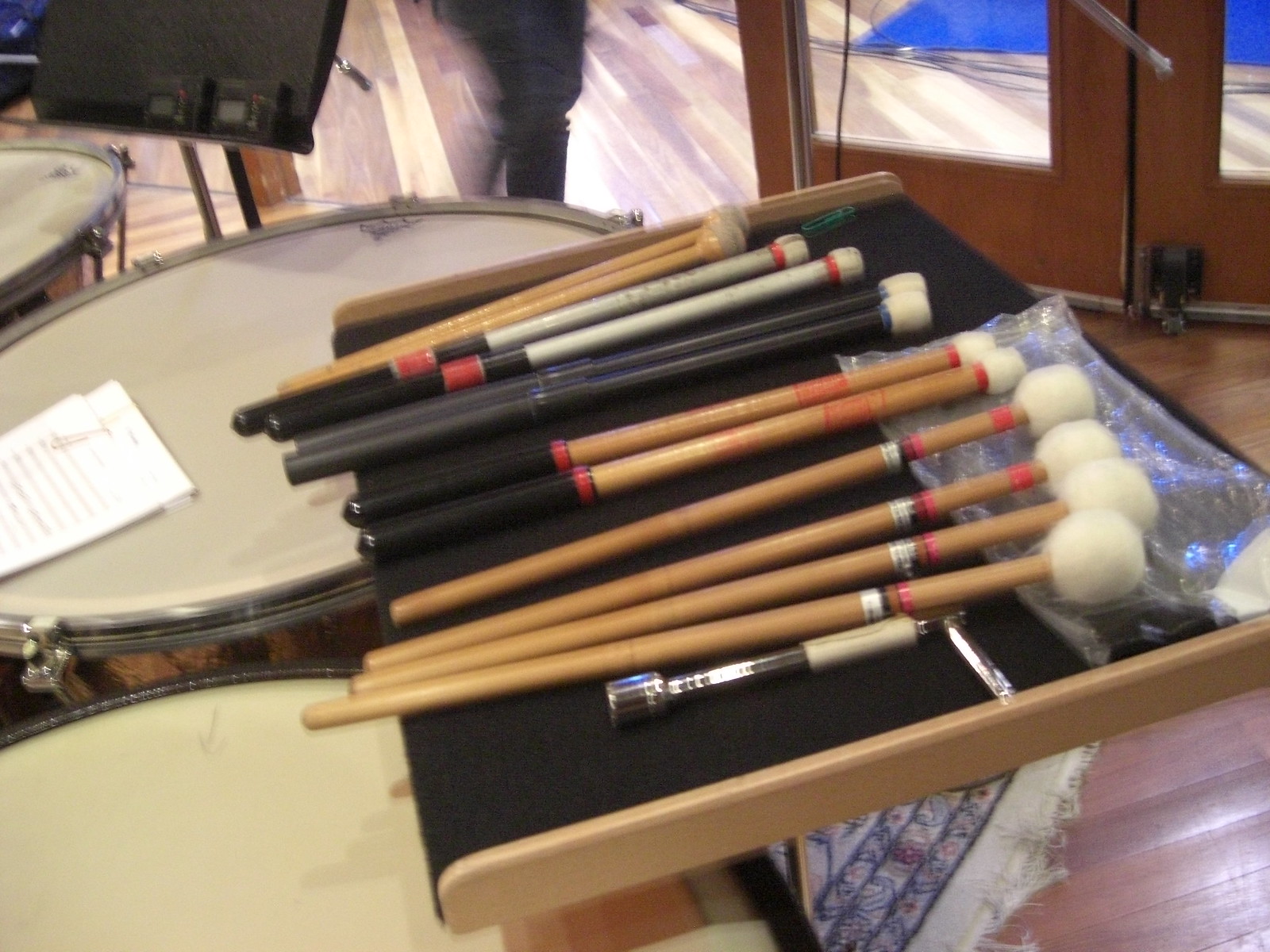The image depicts an indoor setting with a focus on musical instruments, specifically drums and drum accessories. In the upper left corner, part of a drum is visible near a music stand, while below it, a larger drum, white on top and light brown on the bottom, has a piece of paper resting on it. Another drum, with only its top visible, has a holder placed on it containing various drumsticks. The drumsticks are primarily wooden with white tops, but some are also silver, red, and black. Toward the center right-hand side, there is a corner of a carpet on a wooden floor, and in the background, a door with glass panels reveals a glimpse of white and blue beyond it. Despite a slight blur in the photograph, the overall rectangular frame captures the detailed indoor musical setup.